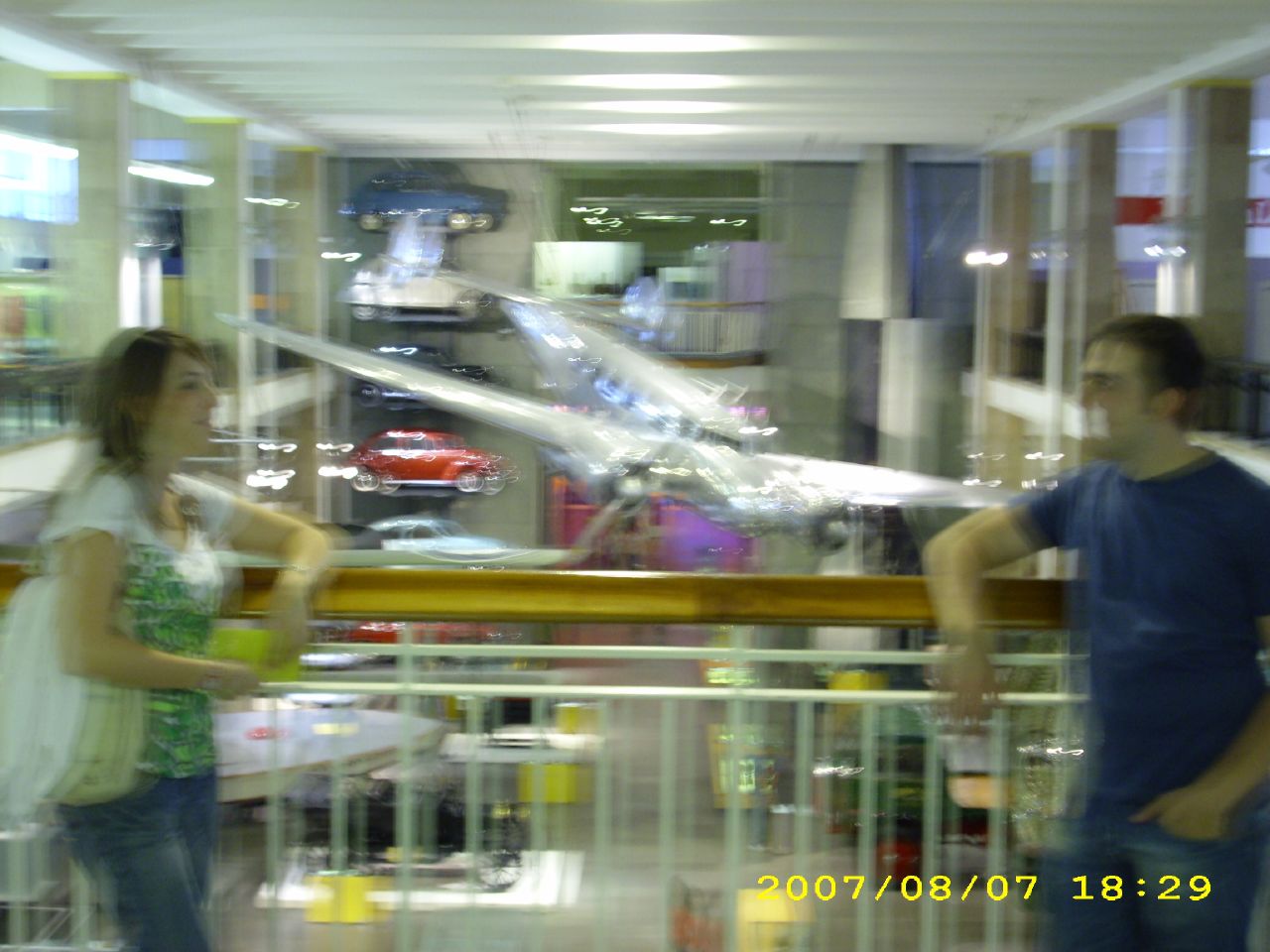In this somewhat blurry photograph, a man and a woman are depicted facing each other, leaning casually with their elbows resting on the white railing of what appears to be a shopping mall. The top of the railing is capped with a horizontal wooden piece. The mall is brightly lit, with fluorescent lights illuminating the scene. In the background, a small airplane is notably on display at their eye level, attracting immediate attention. The photograph captures a bustling atmosphere, with numerous people visible moving about in the background. Behind the woman, additional stores line the mall's interior, their bright lights contributing to the overall illumination. Through the railing, a lower level of the mall can be seen, populated with various items and adding depth to the image.